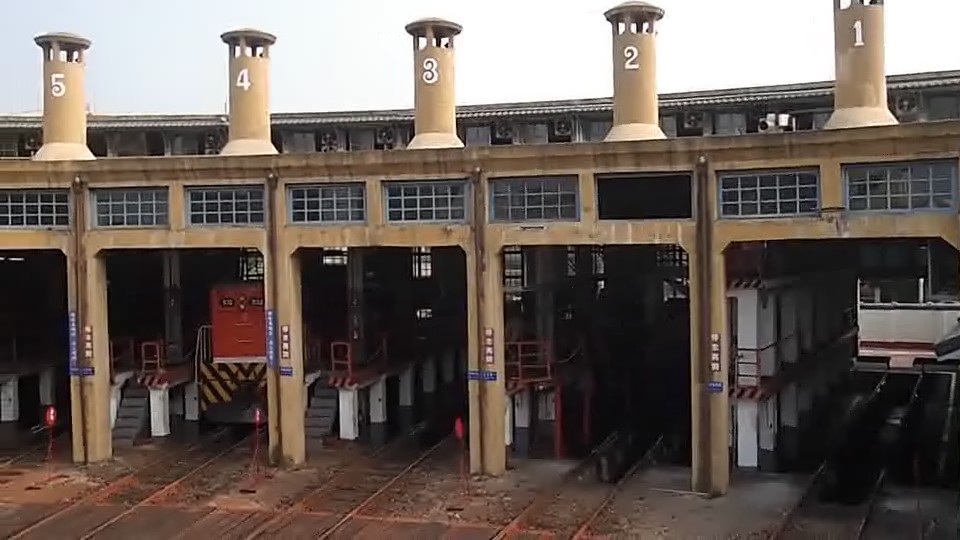The image depicts the famous Changhua Roundhouse in Taiwan, a well-known tourist attraction. The widescreen color photograph showcases the engine shed from a high angle, offering a detailed view of five tunnel-like structures on the face of the building, each with train tracks running underneath. These tunnels, or sheds, are numbered 1 to 5 from right to left in white text on their tan chimneys. Notably, each chimney has a circular umbrella-like cover, except for chimney number 1 on the far right, which is missing this cover.

Above each tunnel entrance is a small, block-style glass window, with one window—third from the left—being broken and empty. The facility also features various elements at the upper part of the building, such as fans in the background.

At the fourth tunnel entrance, a train engine is partially visible. The front half of the engine, basking in light while the back remains in shadow, is painted red with a thin white stripe beneath. The front of the train has yellow and black diagonal hatching on the metal buffers. The ground level beneath the sheds appears old and dirty, featuring a brownish-red color. Sheds numbered 1, 2, 3, and 5 are empty, highlighting the singular presence of a train in shed number 4.